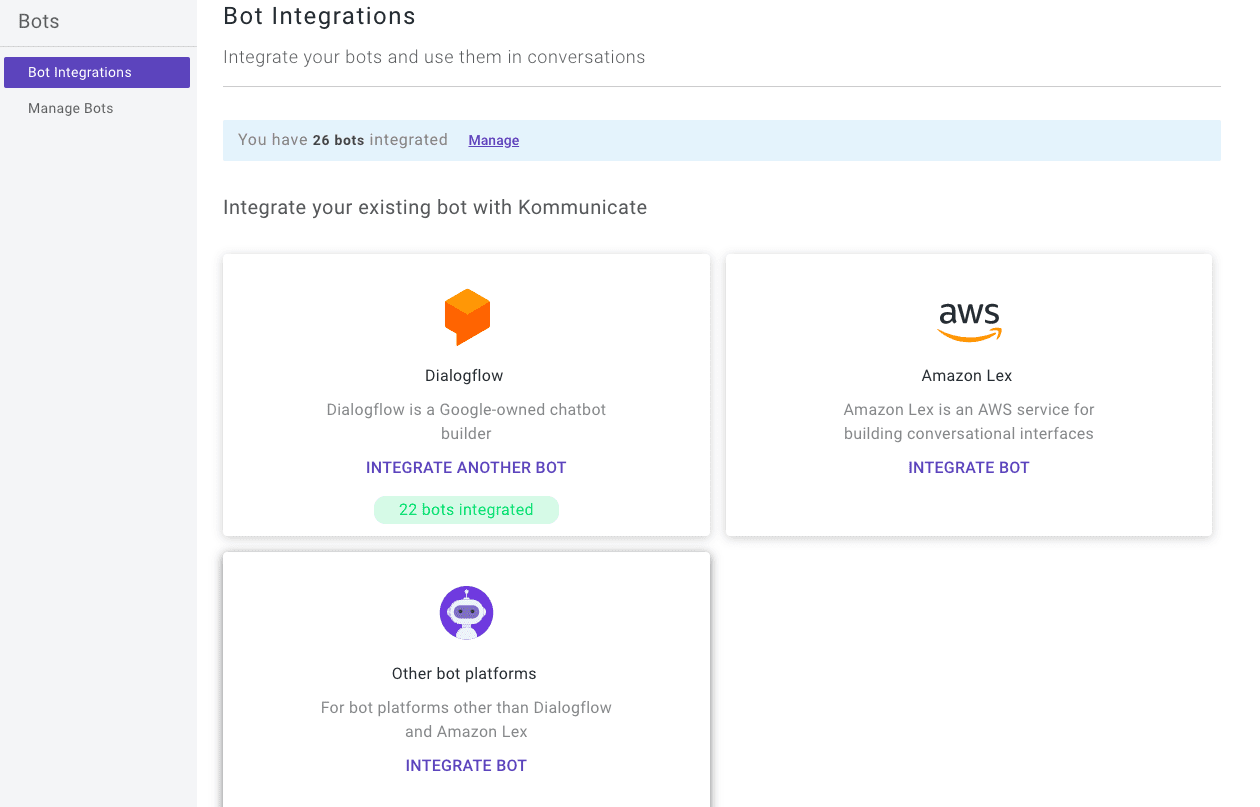The image depicts a user interface for bot integration within a communication platform. In the upper left corner, the section titled "Bot Integration" is prominently displayed. On the left side, a vertical strip contains the word "Bots" at the top, followed by a line, and then "Bot Integrations" in a purple rectangle. Below this, the option "Manage Bots" is listed, all set against a gray background with black font, except for the purple "Bot Integrations" highlight.

The main focus of the image is the "Bot Integrations" section, as it is currently highlighted. This section includes the message, "Integrate your bots and use them in conversations," followed by a dividing line. Below this message is a long blue rectangle which states, "You have 26 bots integrated" and features a "Manage" link in a darker blue with an underline.

The lower part of the image features a white background where users can integrate existing bots with the platform "Kommunicate." This area is divided into two rows, each containing two square tiles for different bots. The first tile is for "Dialogflow," a Google-owned chatbot builder, with the text "Dialogflow is a Google-owned chatbot builder" displayed beneath it. Additionally, there is a button labeled "Integrate another bot" in blue, and another button indicating "22 bots integrated" in light green with dark green font.